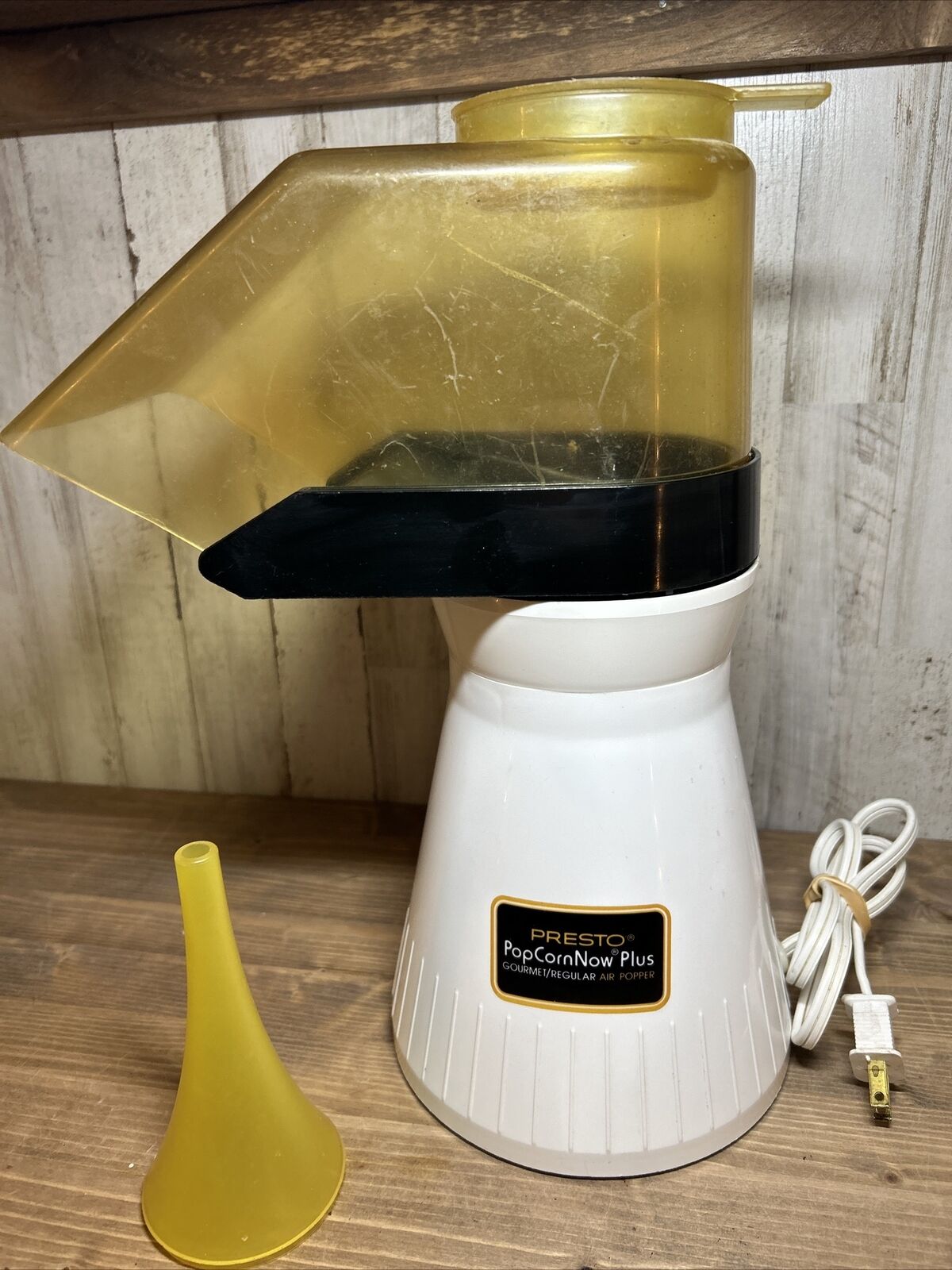This image showcases a vintage Presto Popcorn Now Plus Gourmet Regular Air Popper, likely from the 70s or 80s. The popcorn maker features a white base prominently labeled with its brand and model name. It is topped with a translucent, golden-yellow plastic chute where kernels are inserted. The appliance's cord, a two-pronged plug, is neatly wrapped and secured with a rubber band. An additional accessory, resembling a golden funnel, is placed beside the popper. The setup rests on a wooden surface, with a whitewashed wooden wall and a darker horizontal wood beam as the backdrop, indicating that the popcorn maker is not in use but rather displayed, possibly for sale or as a feature in the photograph.